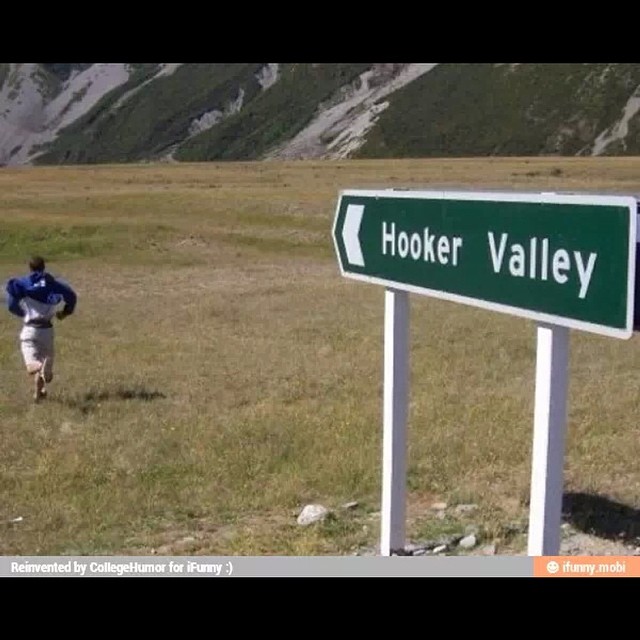This image captures a playful outdoor scene in Hooker Valley, framed by lush grassy meadows and majestic mountains in the backdrop. In the foreground, prominently positioned toward the right, stands a green, rectangular road sign with white text and a left-pointing arrow that reads "Hooker Valley." The sign, mounted on two white poles, contrasts against the tan and green hues of the grass. To the far left of the image, a person dressed in white shorts and a blue jacket is captured mid-run, heading towards the valley with their back turned to the camera. The lower portion of the image includes the humorous text "Reinvented by College Humor for iFunny" and "ifunny.mobi," suggesting a comedic element. The background is dominated by a grassy meadow which transitions into a hillside, with the top fourth of the image revealing the greenish-gray mountains.